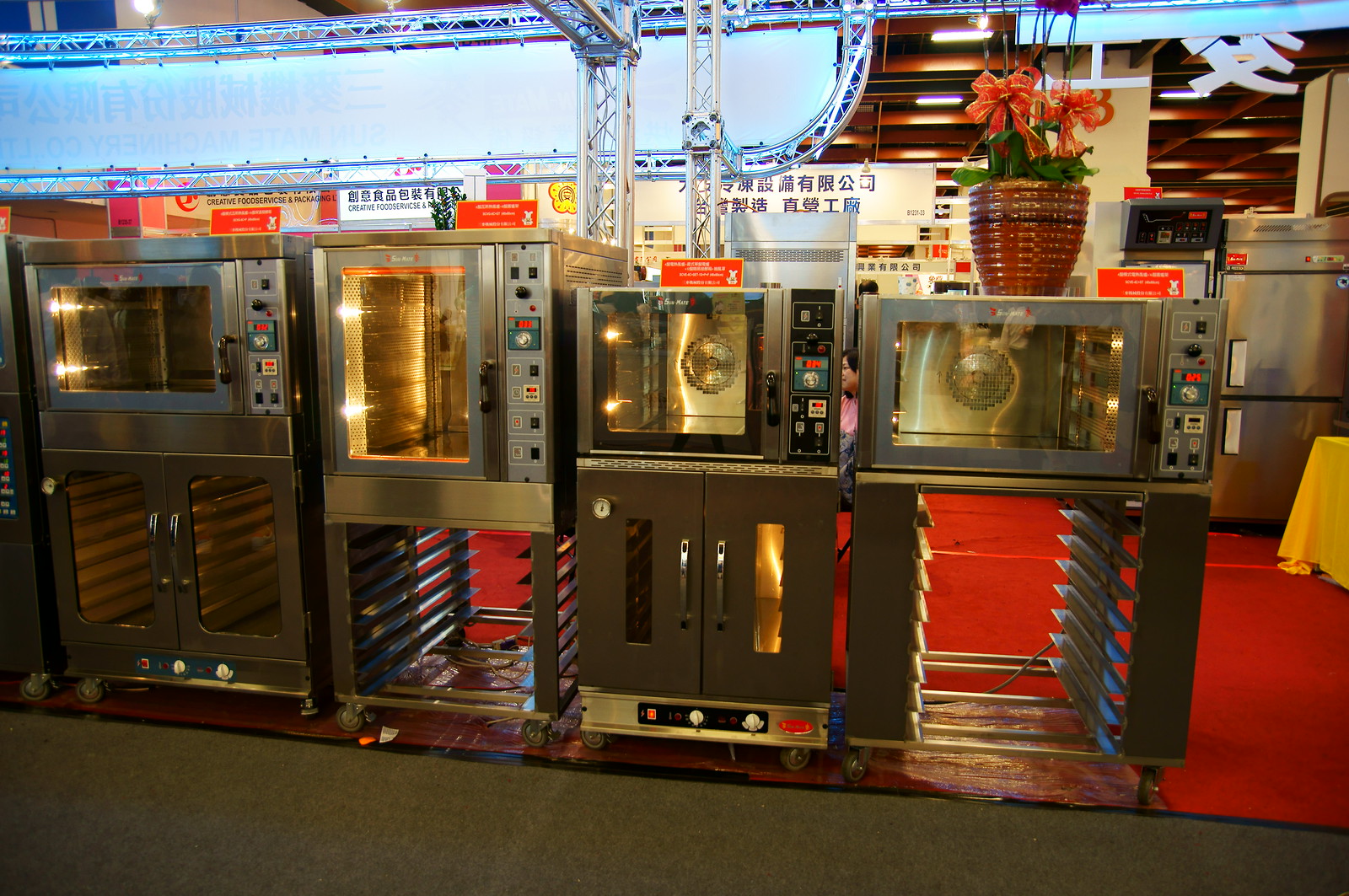The image depicts a spacious Southeast Asian warehouse store, possibly Japanese, featuring industrial and restaurant-style kitchen appliances prominently displayed. The focus of the image is on four large appliances—likely ovens, microwaves, or warming stations—arranged from left to right. Each appliance has distinct features, including dark gray or light gray finishes, multiple doors, black handles, and control buttons on the right-hand side. The appliances have areas for tray placement at the bottom, indicating their use in professional kitchens rather than for consumers. The scene is devoid of people, but the extensive building interior is filled with various appliances in the background, set against a dark gray floor up front and a red floor in the distance. The top of the image features a series of light blue lights illuminating the area. An Asian font and some English text can be seen in the background, hinting at the store's international scope. Additionally, a ceramic vase with ornamental flowers is placed atop the rightmost appliance, adding a decorative touch amid the industrial setting. Metal scaffolding, likely part of a permanent display, can also be seen in the background.